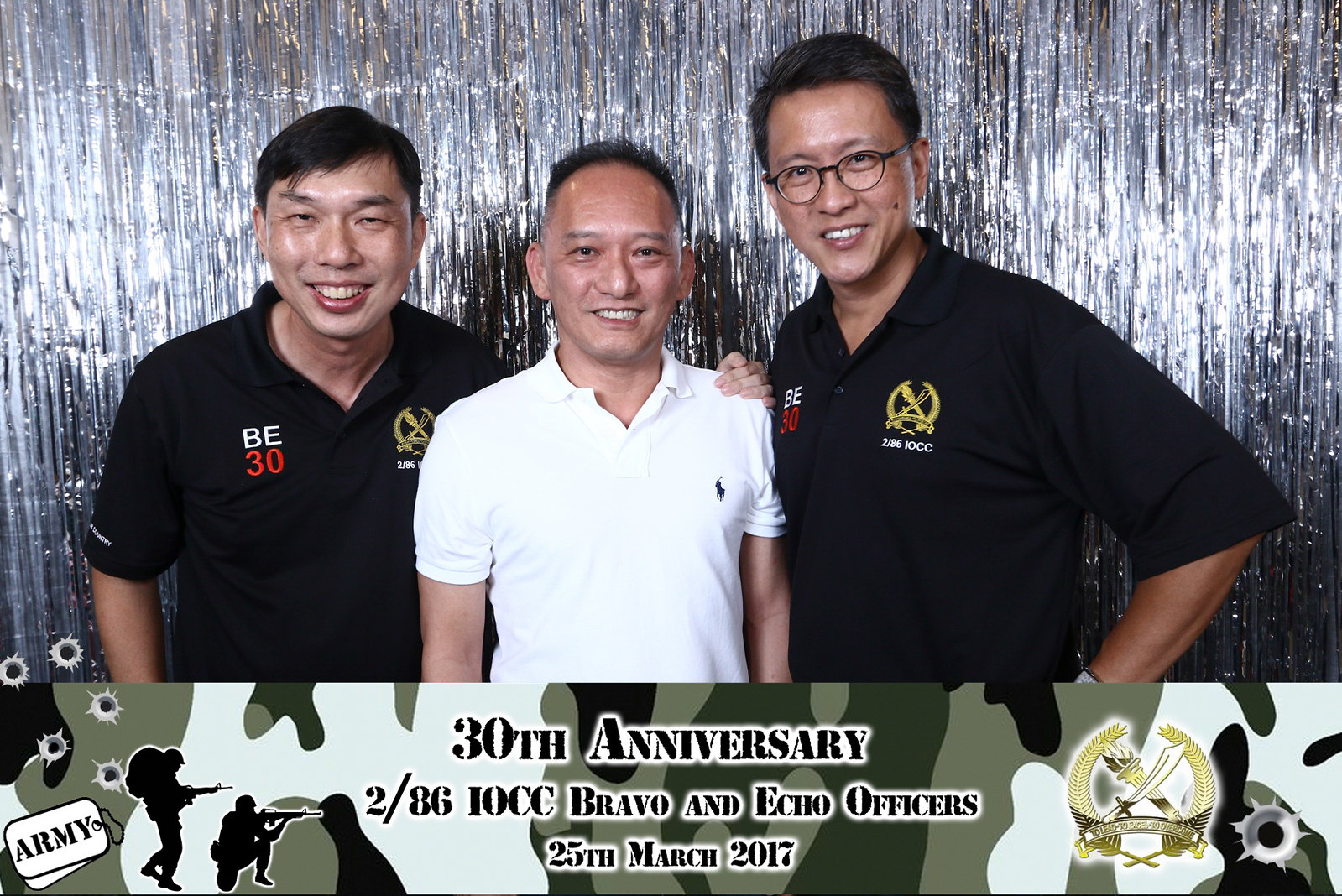In this image, we see three men of Asian descent standing and smiling in front of a silvery, stringy background. The man on the left has short brown hair and is dressed in a black polo shirt featuring the letters "BE" in white, the number "30" in red below it, and a gold emblem on the right chest. The man in the middle wears a white Ralph Lauren polo shirt with a horse logo and has short black hair. The individual on the right, sporting glasses and black hair, is dressed in the same black polo shirt as the man on the left. All three men are smiling warmly. Below them, there's a banner that reads "Army 30th Anniversary, 286 IOCC Bravo and Echo Officers, 25th March 2017" with a camouflage pattern depicting soldiers. The image likely captures a reunion of former service members celebrating their camaraderie and milestone anniversary.